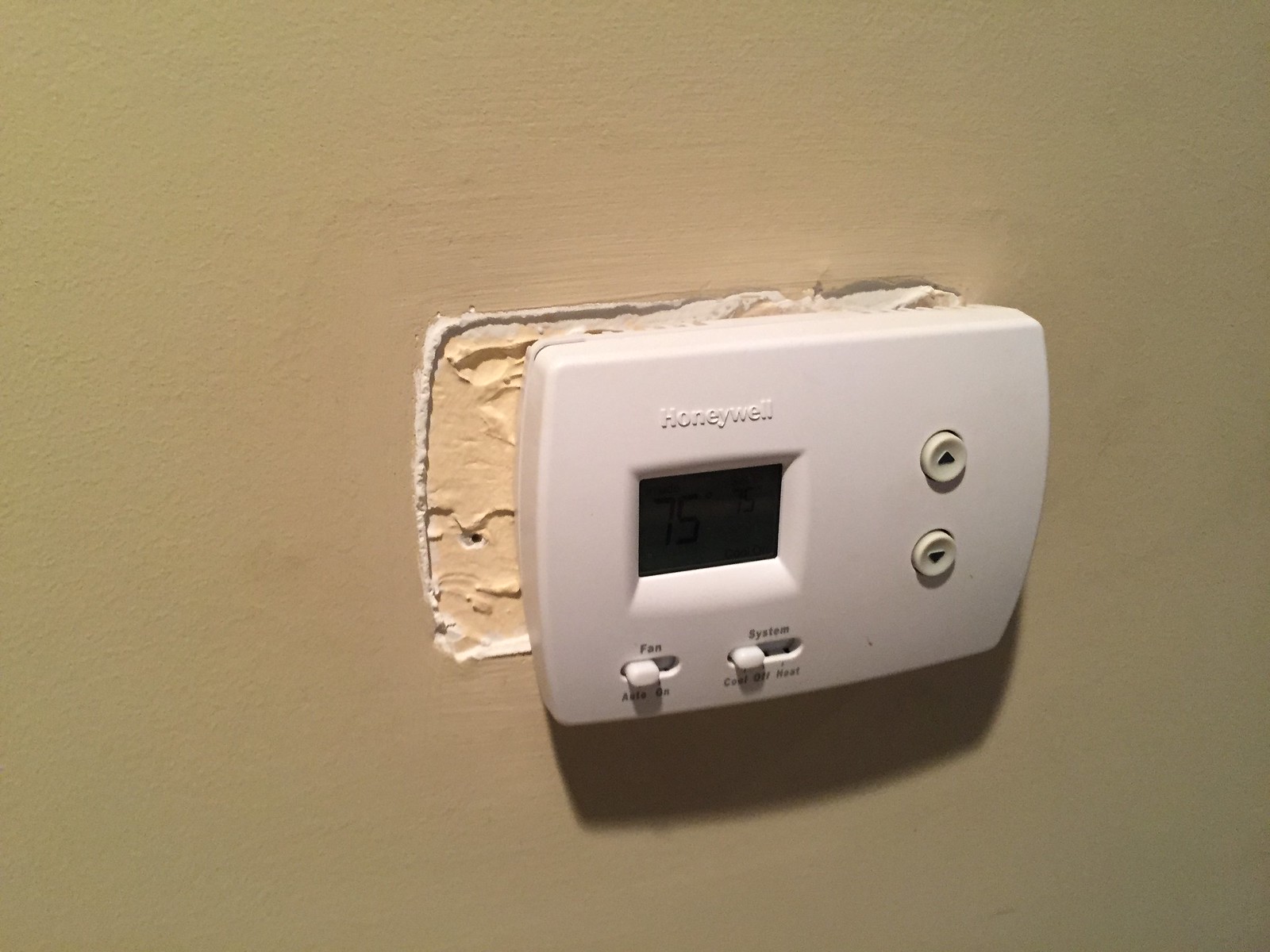A color photograph captures a Honeywell thermostat that has been partially removed from a beige-colored, stucco-textured wall. The plastic outer portion of the thermostat is precariously placed in front of an exposed cavity in the wall, revealing white drywall edges and adhesive residue along the left side of the opening. The thermostat features a digital screen with two buttons positioned below it, and an additional up and down button set on the right side of the front cover. A pronounced shadow extends downward from the plastic cover, emphasizing the gap between the thermostat and the wall.